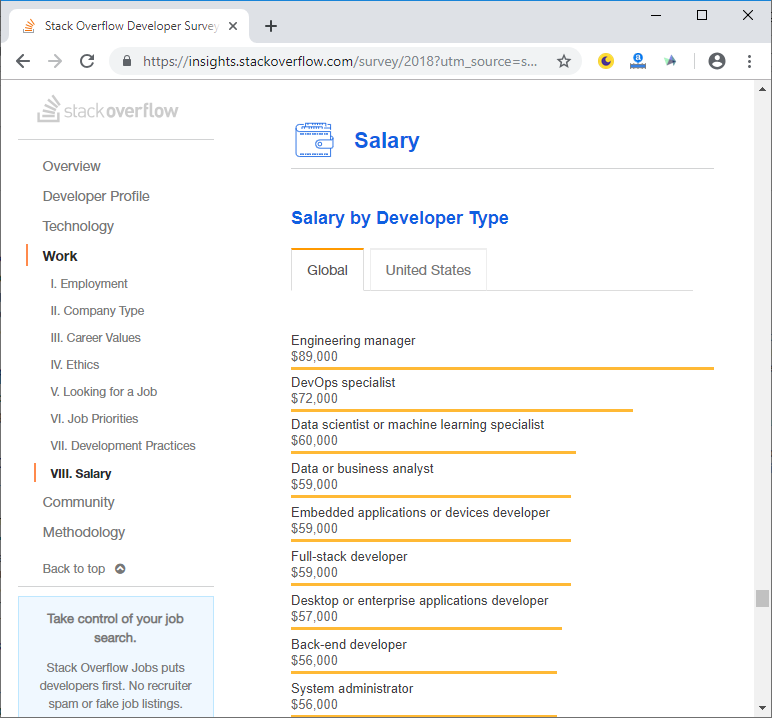A screenshot of a website with a predominantly black-bordered square interface. At the top, there is an emblem depicting a stack of orange, accordion-like books on a black base with the words "Overflow Developer Survey" in front. The emblem features a black “X” on a white background, enclosed in a gray circle. To the right of the "X," there is a black plus sign on the same gray background, continuing across the bar.

On the same row, moving to the right, there are a series of navigation icons: a black left-pointing arrow, a gray right-pointing arrow, and a black refresh button. Below these, there is a search bar with a black lock icon, displaying the URL: "https://insights.stackoverflow.com/survey/2018?utm_source=...". Adjacent to this URL bar, there is a gray star icon, followed by a yellow circle featuring a half-black moon. 

Further to the right, there are two logos: one is a blue circle with a white letter in its center and some white text below, and the other consists of overlapping light blue and gray triangles. A vertical gray line separates these icons from a gray circle that appears to symbolize a person. Following this, there are three gray dots representing more options.

Beneath this navigation bar, the Stack Overflow logo is replicated, accompanied by a more detailed description depicting the stack, with gray papers, and with the words "Stack Overflow" in varying shades of gray. Below this headline is a list formatted with bold section titles. The titles include "Overview," "Developer Profile," "Technology," and "Work," each with a capitalized first letter. To the left of "Work," there’s a short vertical yellow line. Following these titles are bullet points in Roman numerals covering various subsections like "I. Employment" and "II. Company Type."

Towards the bottom, a blue-bordered rectangular box stands out on a light blue background, containing the text "Take control of your job" in bold caps, followed by a promotional message for Stack Overflow Jobs, hinting at the job search focus. Cutting off the tagline, it reads: "Stack Overflow Jobs puts developers first. No recruiter…."

Moving back up to the right side of the screenshot, the heading “Salary” is highlighted in blue, next to an icon resembling a wallet. Beneath this, subheadings read "Salary by Developer Type" followed by two rectangular boxes: "Global" and "United States," separated by a vertical line.

The screenshot further lists various developer roles and their corresponding average salaries, illustrated with horizontal yellow lines. The roles include:
- Engineering Managers: $89,000
- DevOps Specialists: $72,000
- Data Scientists/Machine Learning Specialists: $60,000
- Data/Business Analysts: $59,000
- Embedded Applications/Device Developers: $59,000
- Full-Stack Developers: $59,000 (in gray text)
- Desktop/Enterprise Application Developers: $57,000
- Back-End Developers: $56,000
- Systems Administrators: $56,000

Each salary is prefixed by a dollar sign and formatted consistently across the list, concluding with horizontal yellow lines indicating progression from one salary tier to the next.

This detailed description captures the entirety of the visual elements, layout, and content within the screenshot.